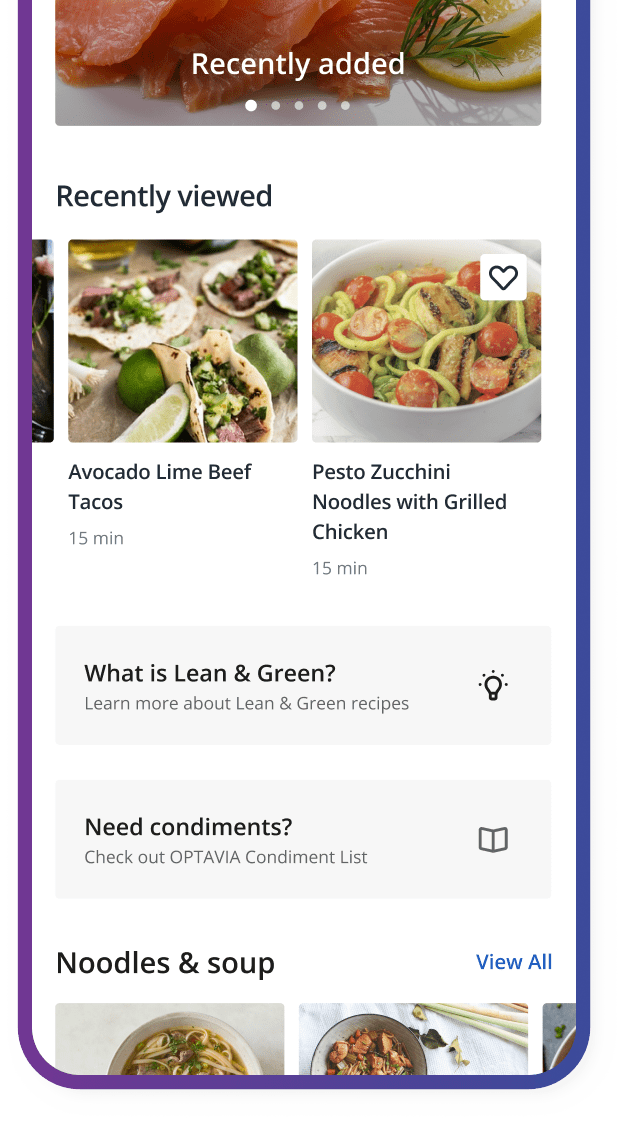This image displays a variety of culinary dishes and associated descriptions against a predominantly white background. In the top-left corner, there's a blue notification banner indicating a recently added recipe labeled as "Tuna and Lemon." Adjacent to it, a black test indicates "Recently Viewed" with a specific highlight on "Avocado Lime Beef Tacos." Below this, a bowl is presented with a label "Pesto Zucchini Noodles with Grilled Chicken, 15 minutes."

At the center of the image, there's information about "Lean and Green" recipes, encouraging viewers to learn more about these nutritious options. Next to this, an icon of a bulb suggests additional helpful tips or ideas. Another section advocates checking out the "Octavia Condiment List," suited for those needing guidance on condiments.

Toward the bottom left, an open book graphic includes the description "Noodles and Soup," showing what seems to be a noodle soup on the left and another type of soup on the right, with chopsticks visibly placed in the image. The smartphone depicted has a blue edge on the right that transitions to a purple edge on the left, creating a subtle gradient effect.